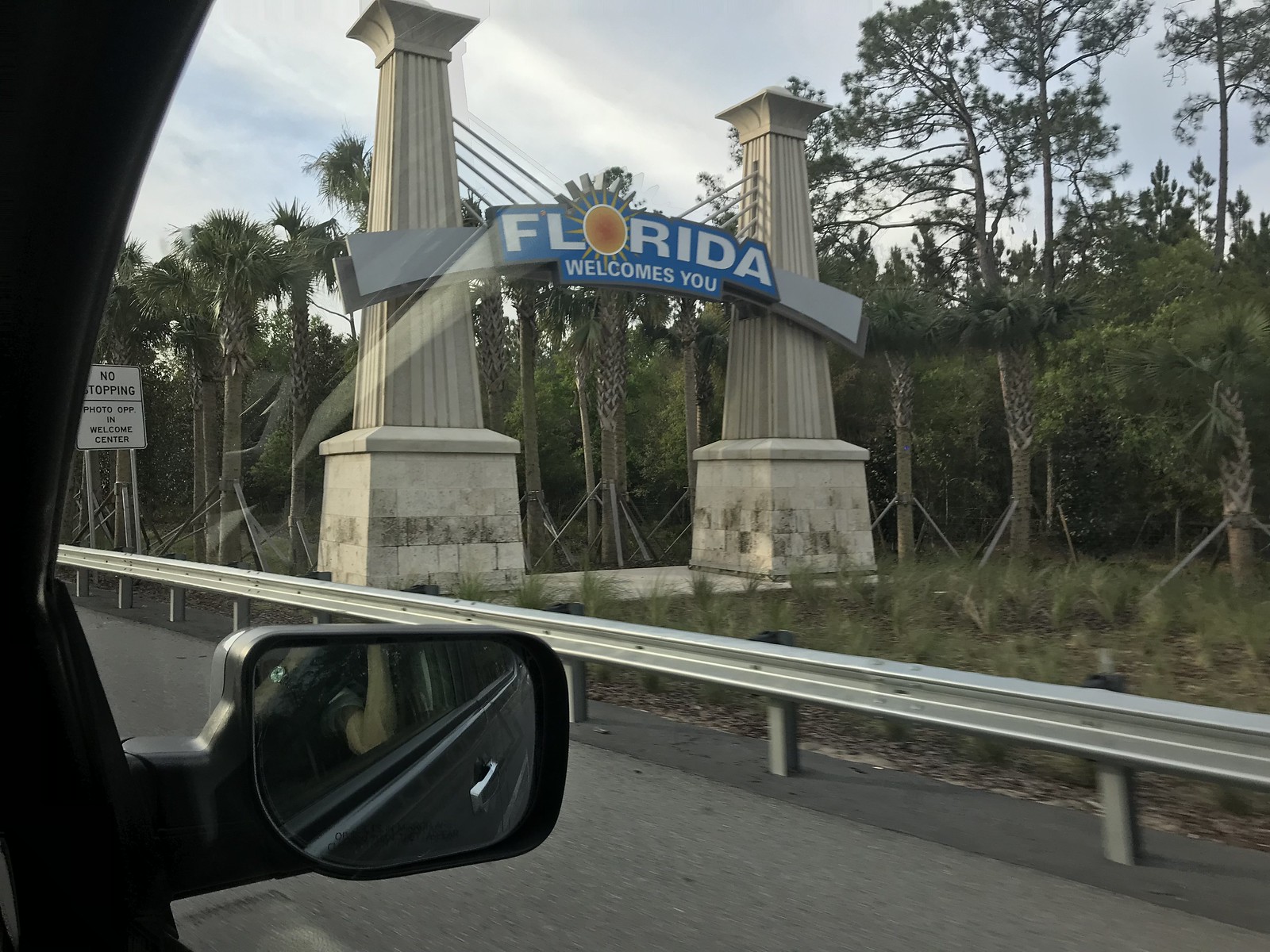Captured from inside a vehicle, this image showcases a vibrant "Florida Welcomes You" sign, designed as a striking monument with two tall pillars supporting a horizontal board. The sign, resplendent in blue and orange hues, features a sun as the 'O' in "Florida," adding a warm and inviting touch. In the foreground, the picture reveals the vehicle's rearview or side mirror, along with the arm of the person taking the photo, emphasizing the on-the-go nature of the moment. On the left side of the image, a street sign is visible, clearly stating "No Stopping - Photo Op in the Welcome Center," reflecting the rules for travelers eager to capture their arrival. The background is adorned with lush palm trees, enhancing the tropical Floridian atmosphere.